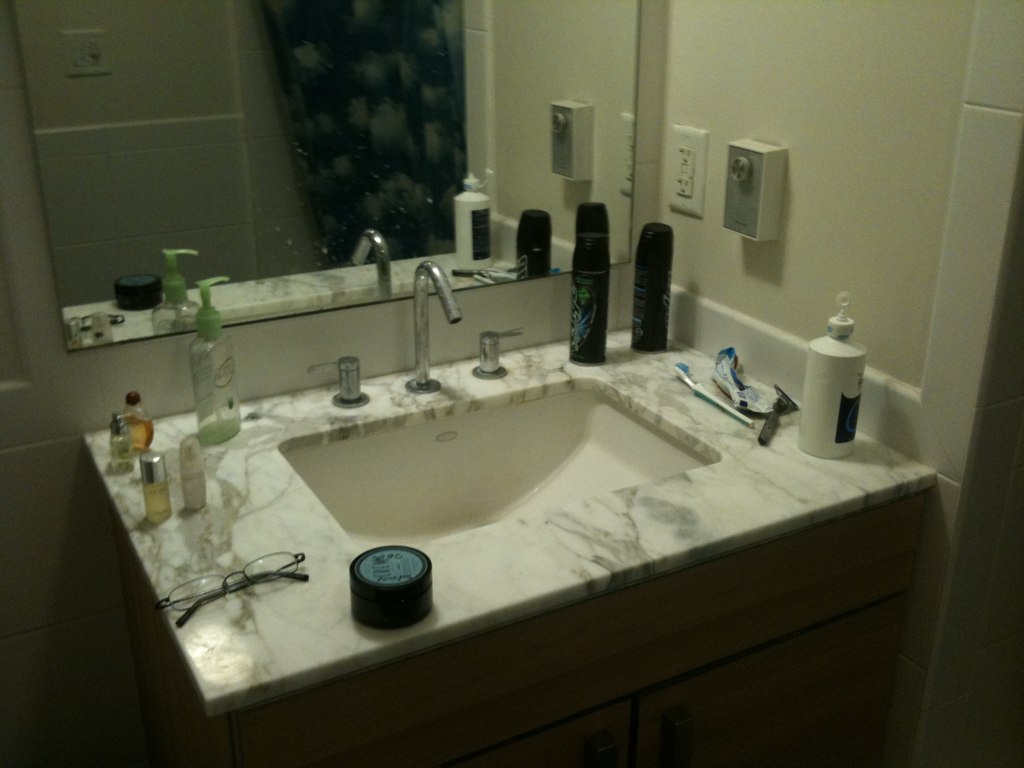This dimly lit and slightly blurry photograph features a bathroom sink, suggesting it was captured in low lighting conditions. The visible portion of the sink's countertop appears to be made of white marble with black veining. Centrally positioned at the front of the sink is a black circular object, flanked on one side by a pair of eyeglasses. In the left corner of the sink countertop are four small bottles, resembling perfume bottles, containing liquids of varying hues—some darker, some yellow, and one with a golden tint. Neighboring these bottles is a container with a green lid, likely soap. The sink hardware, including the hot and cold water taps and the spout, is silver in color. On the right corner of the countertop sits two black bottles, a toothbrush, a visibly squeezed tube of toothpaste, and a bottle of saline solution. Additionally, the wall behind the sink features two electrical outlets. The overall setting gives the impression of a hotel bathroom. The photograph also captures the edge of a mirror above the sink, though the reflection in the mirror is not visible.